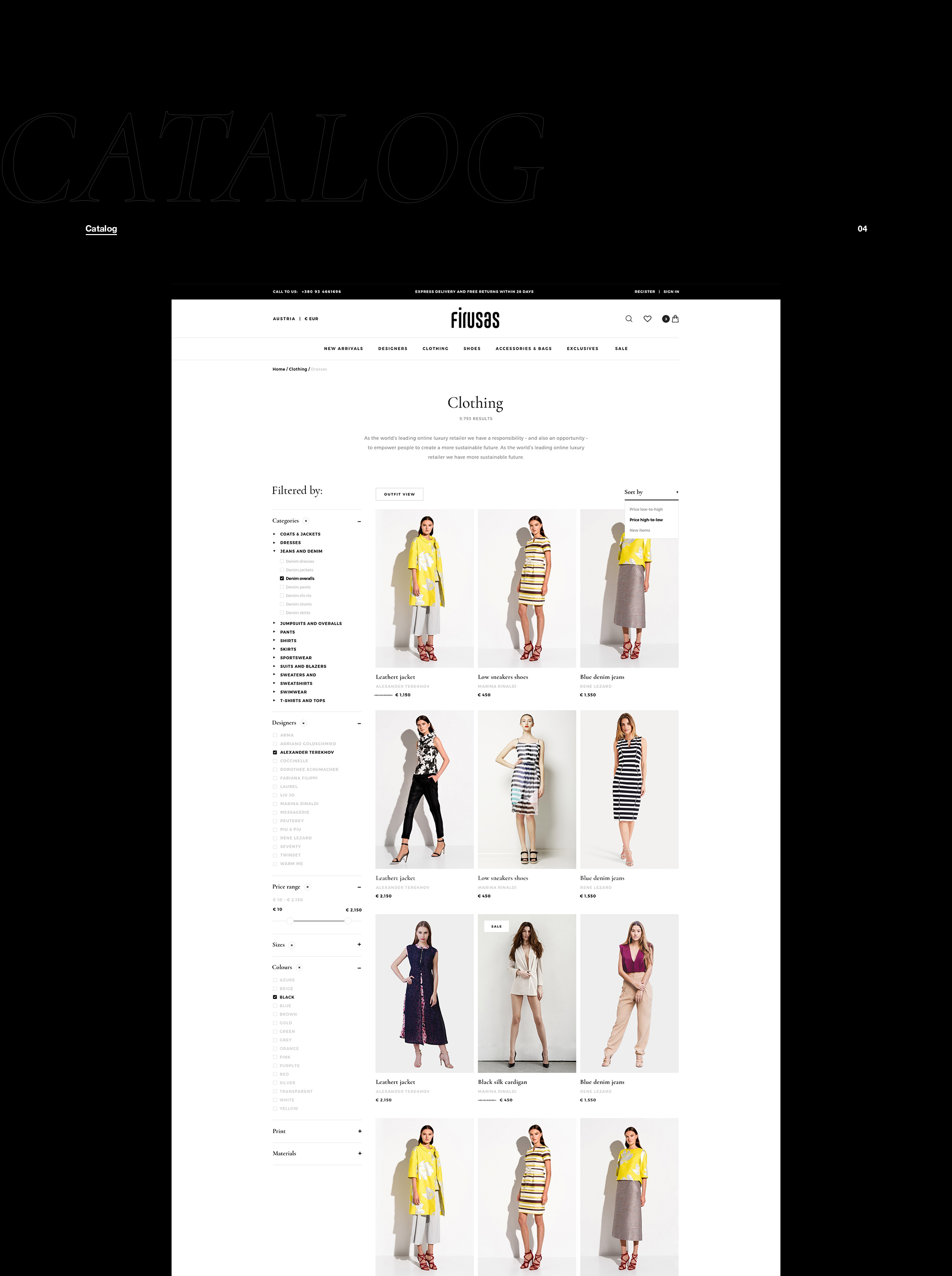The image features a black background with a vertically elongated format. Positioned slightly down on the left side in white text is the word "Catalog." Central to the image, there is a white rectangle containing the text "FIRUSAS." Due to low resolution, the text above "FIRUSAS" is illegible. Below this, in smaller text, there are some partially readable words: "DECI-CNE-SEAS, clothing," followed by some obscured lines, with the visible phrases including "accessories" and "something exclusive, sale." Large text further down reads "clothing."

Beneath these headings, there is a paragraph of text that is too blurred to decipher. Below the paragraph, there are three rows of images displaying clothing items, and an additional fourth row is visible. Navigational options are present on the left side, listing filters such as "Filter By," "Categories," and specific categories of clothing including "Coats and Jackets," "Jeans and Denim," "Jumpsuits and Overalls," "Pants," and what appear to be "Shirts or Skirts" and "Sportswear."